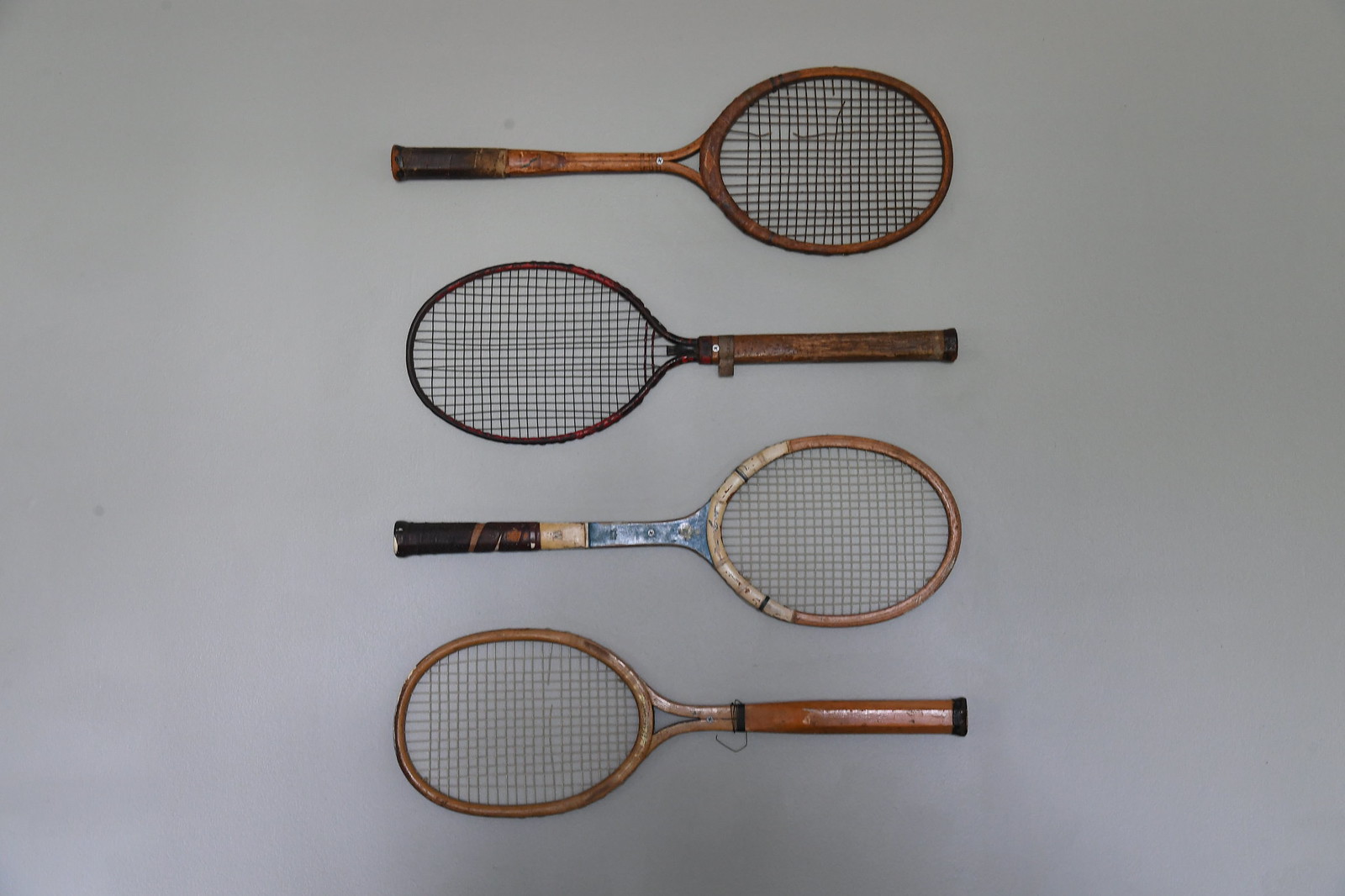This image features four antique tennis rackets lined up vertically on a blank light gray background, each with distinctive features. At the top, the first racket is made of light brown wood with a darker brown handle oriented to the left. It has numerous broken strings. Below it, the second racket is quite similar but mirrors the first with the handle facing right. This handle is slightly lighter in color and features a brown strap near the top. The third racket, with its handle facing left, stands out with a metal section connecting the strings to the handle, which is wrapped in black leather. The head of this racket has light brown and yellow layers. The bottom racket has its handle facing right, adorned with black piping and a loose black string around the handle’s top. There are noticeable wear marks and multiple broken strings within the racket's head. All rackets highlight an aged, antique appearance, contributing to the vintage charm of the composition.